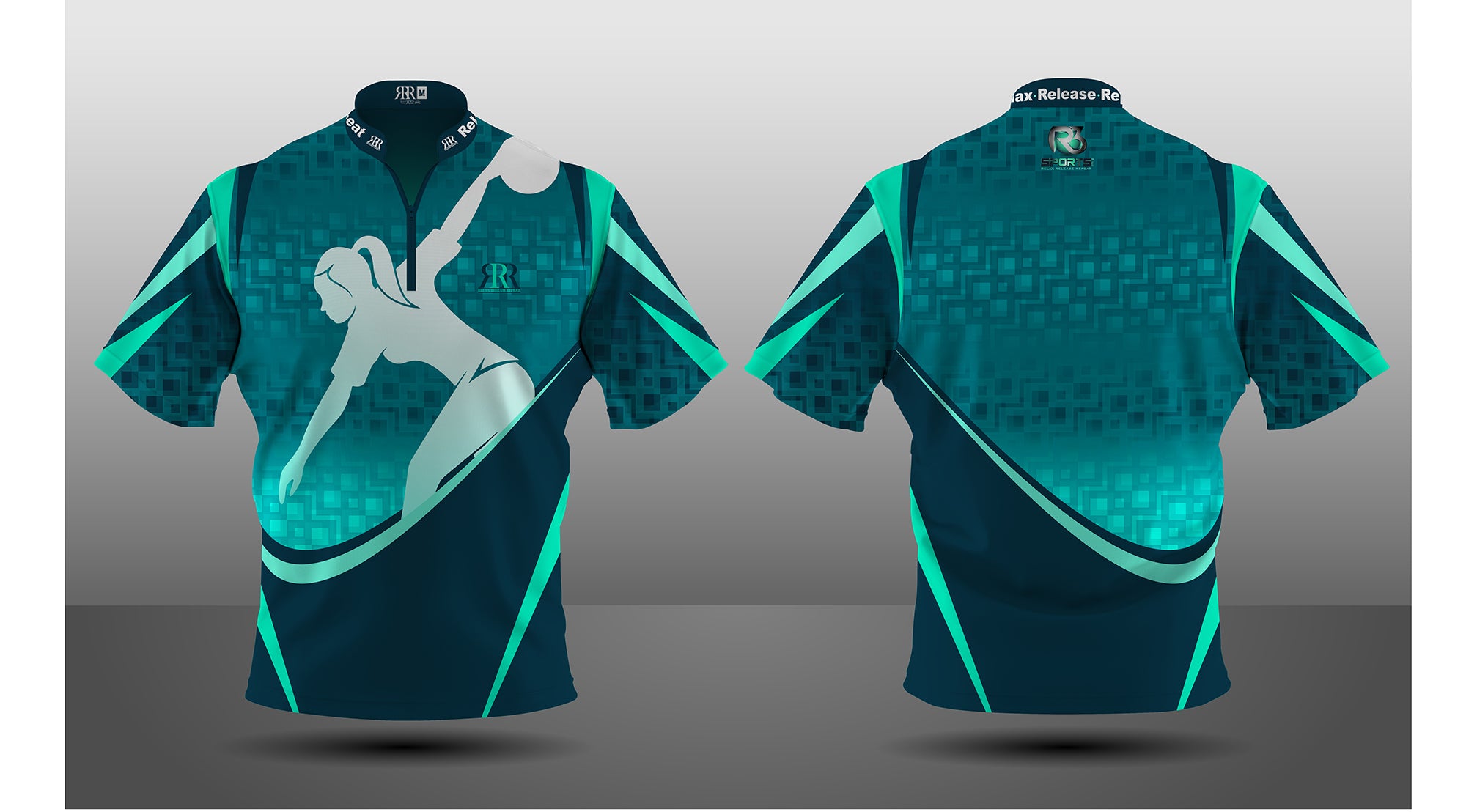In this computer-generated graphic, two stylized short-sleeved shirts are displayed side by side against a gray background, with their shadows cast in a darker gray hue, creating the illusion that the garments are floating. The shirt on the left shows the front side, primarily featuring a teal color with a geometric pattern of lighter squares and diamond shapes, lending it a futuristic appearance. Various curves and lines in a lighter teal accentuate the design, which transitions to a darker green-teal at the bottom. The front of the shirt also includes an emblem on the upper right breast, depicting a silhouette of a woman with a ponytail poised to throw or bowl, rendered in a lighter teal. The black collar has white text that is difficult to discern. The shirt on the right reveals the back, continuing the geometric pattern but without the female figure or emblem. On this side, the black collar bears the partially legible word “release”. Both shirts feature a blend of dark blue and turquoise swaths on the shoulders and lower areas, enhancing their dynamic, sporty look.